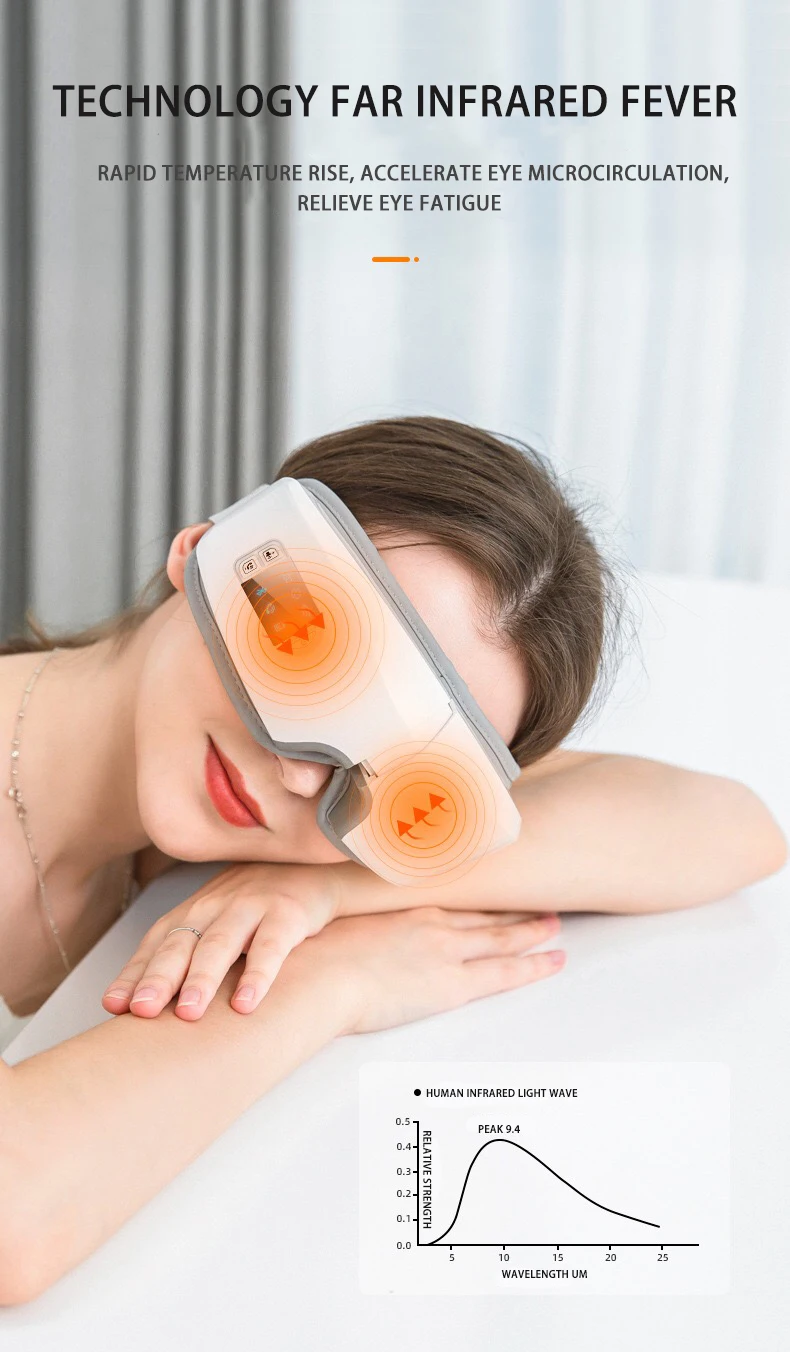The image showcases a fair-skinned young woman with brown hair, wearing red lipstick and a thin necklace. She rests her head on her arms, lying on a white pillow or surface. Over her eyes, she wears a distinctive pair of white eye patches or goggles featuring arrows pointing toward the center from either side, and orange circles over the eyes. The background is predominantly gray with a gray curtain and a white vertical blind behind her. The top of the image contains bold black text stating, "Technology Far Infrared Fever," followed by smaller text that reads, "Rapid Temperature Rise, Accelerate Eye Microcirculation, Relieve Eye Fatigue." At the bottom right is a black line graph labeled "Human Infrared Light Wave," with "Relative Strength" on the y-axis and "Wavelength Micrometers" on the x-axis. The graph peaks at 9.4 and spans from 1 to 25 micrometers. The image is a vertical rectangle, approximately two and a half times taller than it is wide.